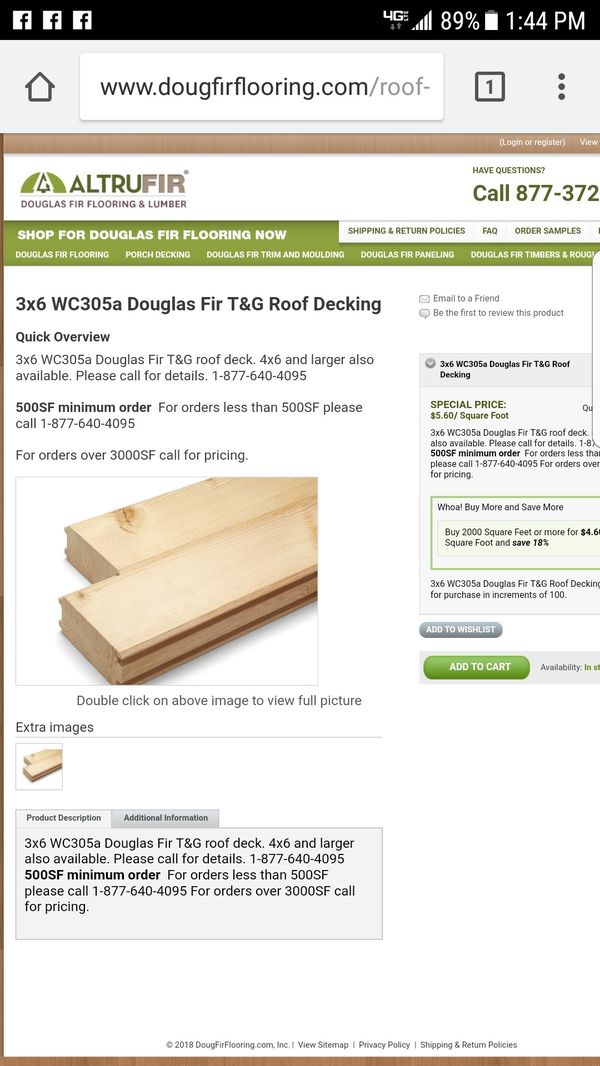The image is a rectangular screenshot from a mobile browser, oriented vertically. The top section of the image has a black border containing three Facebook icons on the far left, a 4G signal indicator with full bars, a battery icon showing 89% charge, and the time displayed as 1:44 p.m. The browser's address bar shows a URL (doorfurflooring.com/roof) with a home icon to its left, a tab indicator with the number 1, and a three-dot vertical menu on the far right. 

Beneath this, there is a brown border displaying the text "All True for Douglas Fir Flooring and Lumber" aligned to the center with a number on the right. A green border separates this section from the rest of the webpage content below. 

The main content area promotes various Douglas Fir products, including a call to action saying "Shop for Douglas Fir Flooring Now." It lists items such as Douglas Fir Flooring, Porch Decking, Douglas Fir Trim and Molding, Douglas Fir Paneling, and Douglas Fir Trim and Rough. Accompanying these descriptions is an image showing Douglas Fir lumber, which appears to include some tongue and groove boards along with detailed descriptions of the available products.